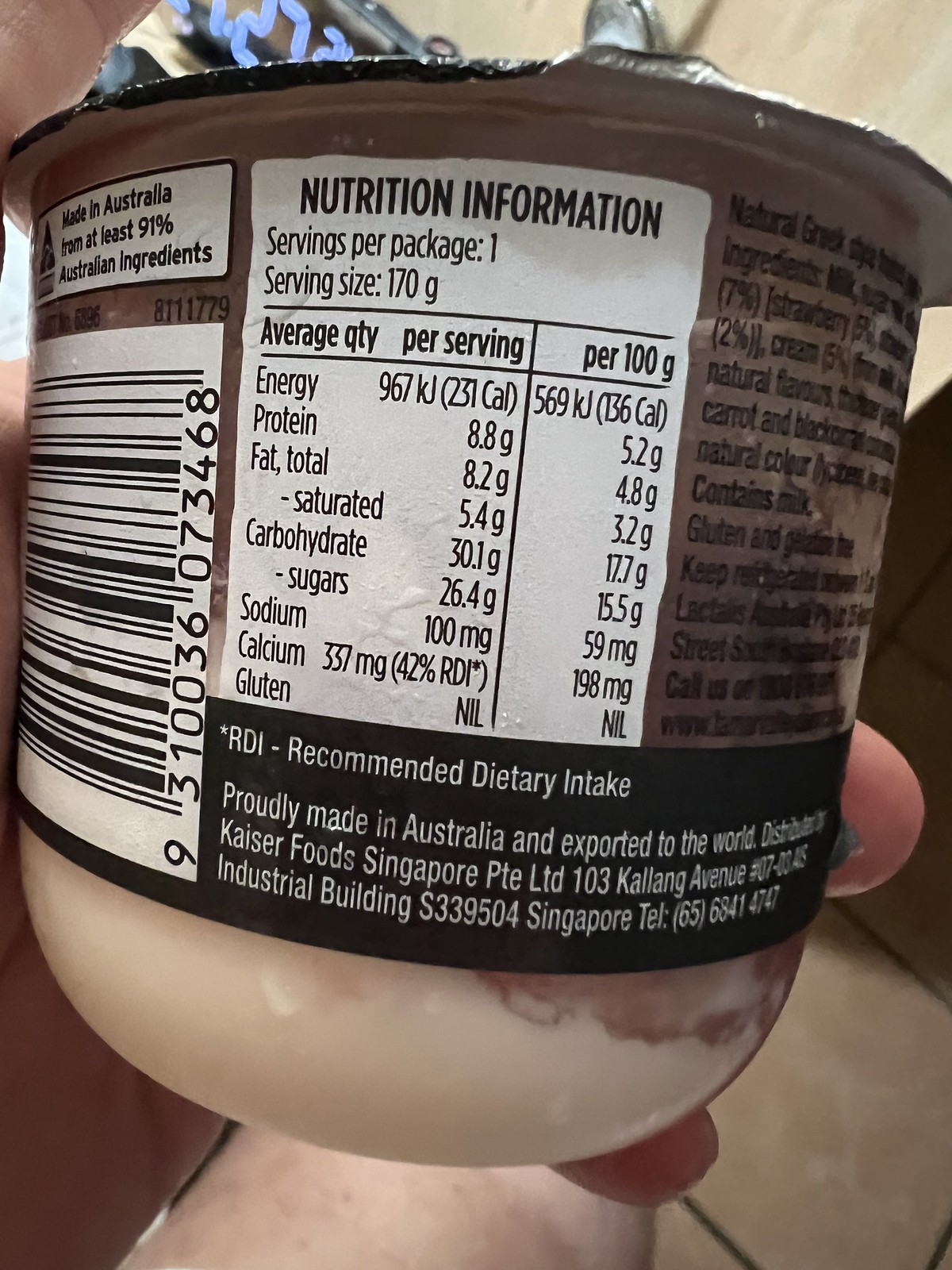The image captures a close-up of an individual-sized yogurt container being held by a person's hand, angled towards the camera to display its nutritional information. The container is grasped in the left hand, with two fingertips visible around its edge, and the person appears to be sitting as their left thigh is partly visible in the frame, atop a light tan tiled floor with dark grout lines.

The yogurt, identifiable by the typical container shape and remaining contents, prominently features a label stating "Made in Australia from at least 91% Australian ingredients" along with a vertical barcode (9310036073468). The foil top seems to be either partially peeled back or reflecting a nearby digital display, possibly a clock or stove top, seen in the top left of the image.

The nutritional information on the container lists: 
- Servings per package: 1
- Serving size: 170 grams
- Energy: 967 kJ (231 kcal) per serving, 569 kJ (136 kcal) per 100 grams
- Protein: 8.8 grams per serving, 5.2 grams per 100 grams
- Fat total: 8.2 grams per serving, 4.8 grams per 100 grams
- Saturated fat: 5.4 grams per serving, 3.2 grams per 100 grams
- Carbohydrates: 30.1 grams per serving, 17.7 grams per 100 grams
- Sugars: 26.4 grams per serving, 15.5 grams per 100 grams
- Sodium: 100 milligrams per serving, 59 milligrams per 100 grams
- Calcium: 337 milligrams per serving, which is 42% of the recommended daily intake
- Gluten: NIL

The text on the label indicates the yogurt is distributed by Kaiser Foods Singapore, PTE, Ltd., located at 103 Colling Avenue, Industrial Building 07, Singapore 339504, with contact number 656 841 4747. The detailed nutrition and distribution information suggest a clear emphasis on the product's Australian origin and global distribution.